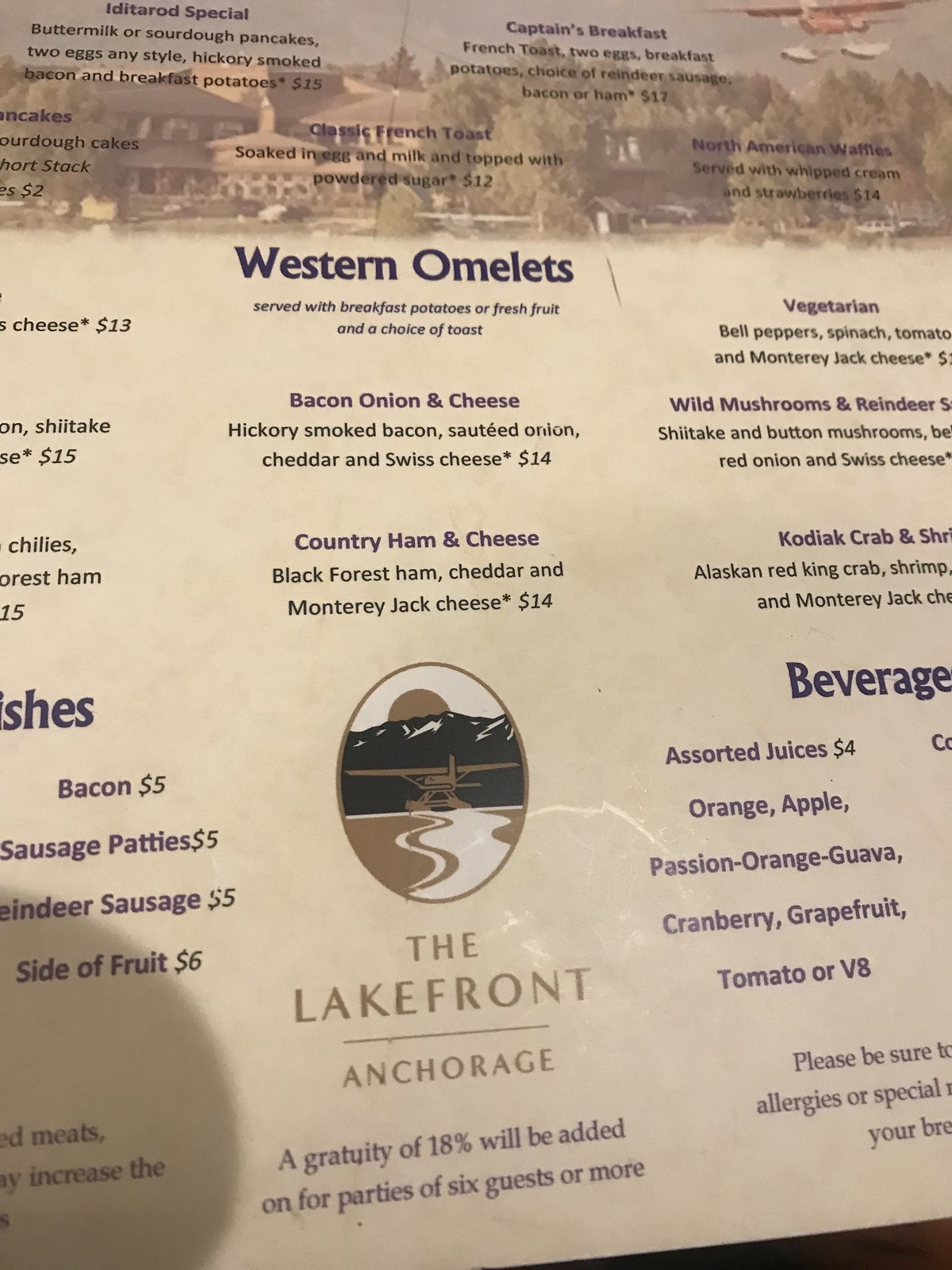This photograph captures a menu in a portrait orientation, which is somewhat inefficient as it truncates a significant portion of the menu, revealing only a selection of items. The menu's bottom 75% features a tan background with blue and black lettering, making it visually distinct. The upper section of the menu depicts a semi-transparent scenic illustration of a large house, a couple of trees, and it overlays some menu items. 

Prominently displayed in large blue letters at the upper center, the menu highlights "Western Omelets," offering options such as bacon, onion, and cheese, as well as country ham and cheese. Just below this, there is a label with a brown border featuring black mountains, a brown lake or river, and a brown sunrise, and it reads "Lakefront Anchorage" in brown text. This section also lists various beverages, including assorted juices.

Moving upwards, the menu lists other omelet options such as a vegetarian omelet, wild mushroom, reindeer, and Kodiak crab. Additional items, albeit hard to discern due to the scenic background, include dishes named bacon, sausage patty, reindeer sausage, cider, fruit, and possibly some specials written in black lettering. The overall composition of the menu is detailed but somewhat cluttered due to the overlapping of the scenic elements with the text.